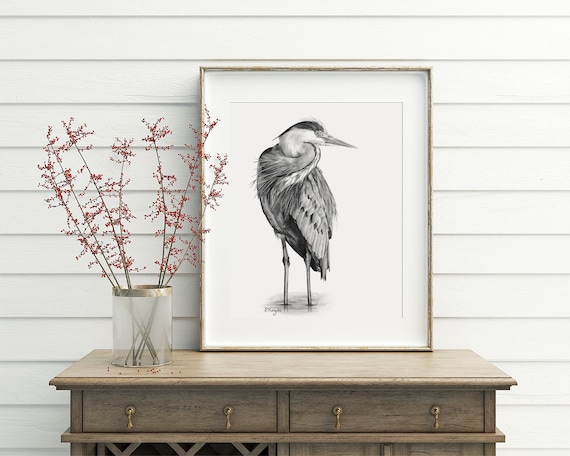The image is a detailed black and white pencil drawing of a bird, with the body facing the camera and the head turned to the left. The bird's head is black, its face and neck are white, and its body features a blend of gray and black. The wings are a mix of black and white, and it has two scrawny legs, suggesting it is standing in rippling water. The artwork is displayed in a light brown, thin frame with a white matting, placed atop a rustic, light brown wooden desk with two drawers, each adorned with brass handles. Standing to the left of the framed art is a frosted clear vase with a gold rim, filled with twigs that bear red berries. The setting includes a white wall with line detailing, creating a harmonious background with the medium brown desk and its minimalist décor.